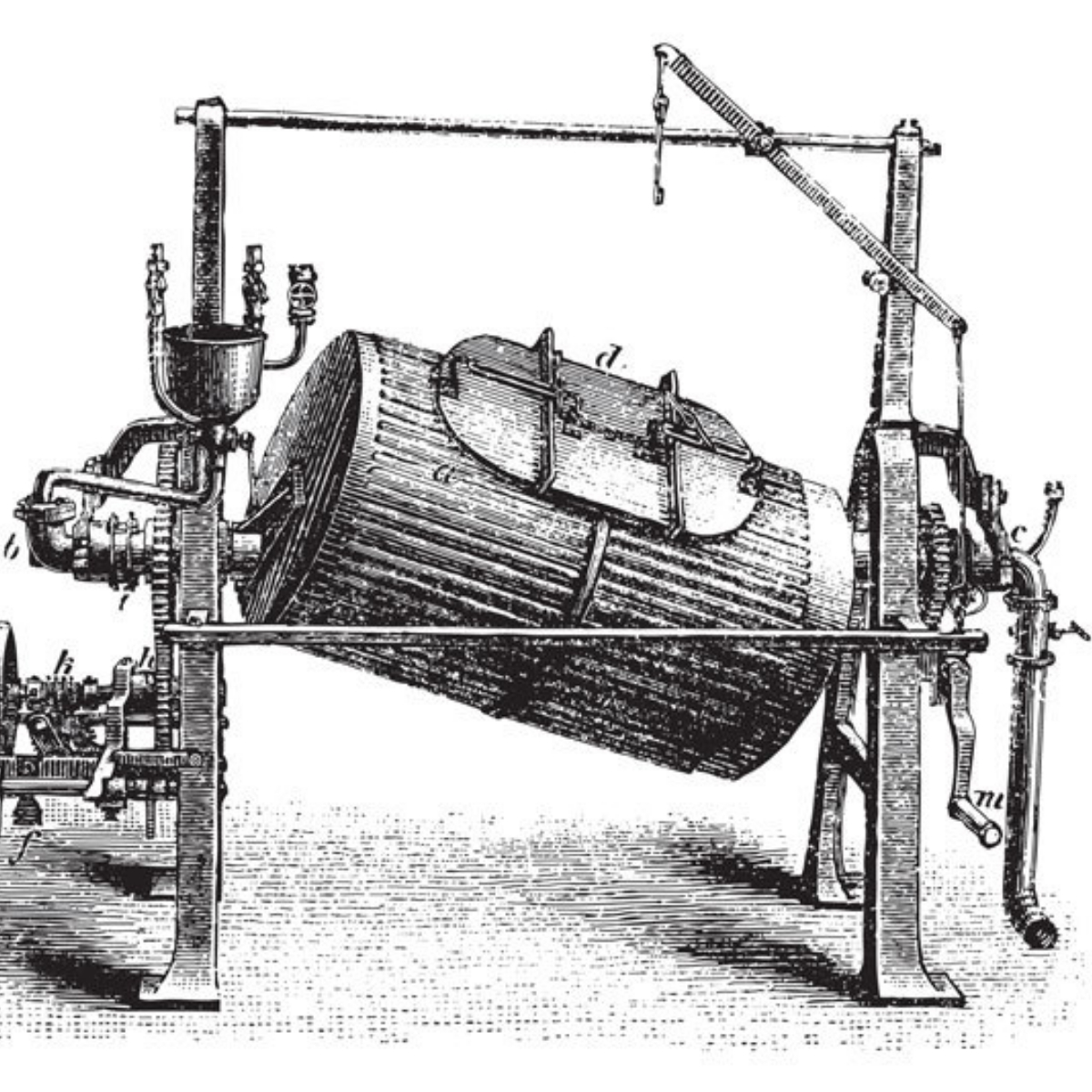This detailed illustration features a black and white pencil line drawing of a mechanical device against a white background. The device consists of a large, sturdy frame supported by two stands, each with dual legs converging at the top into a single arm. These legs are connected by a round metal rod both at the top and midway down. Centrally placed within this frame is a substantial cylindrical component, identifiable by its pronounced ridges and an oval-shaped door, marked with the letter "D," situated on its upward-tilting side. This cylinder appears to function on a horizontal plane but is noticeably tilted to the right. A large tube enters and exits this cylinder through gaps in the frame, creating a complex pattern of connections.

To the right of the cylinder, a crank is attached to a cog mechanism, suggesting a manual or mechanical operation. Additional bars and smaller metal pieces extend from the right side of the frame, including a metal pipe with an open end at the bottom. A bar ascends from this pipe, extending upward and arching towards the central top bar of the structure, from which a small chain hangs. The intricate web of hooks, wires, and mechanical parts propping up the cylinder adds to the machine's complexity, evoking the look of an engineered prototype or a conceptual rendering rather than a fully realized, purpose-defined machine.